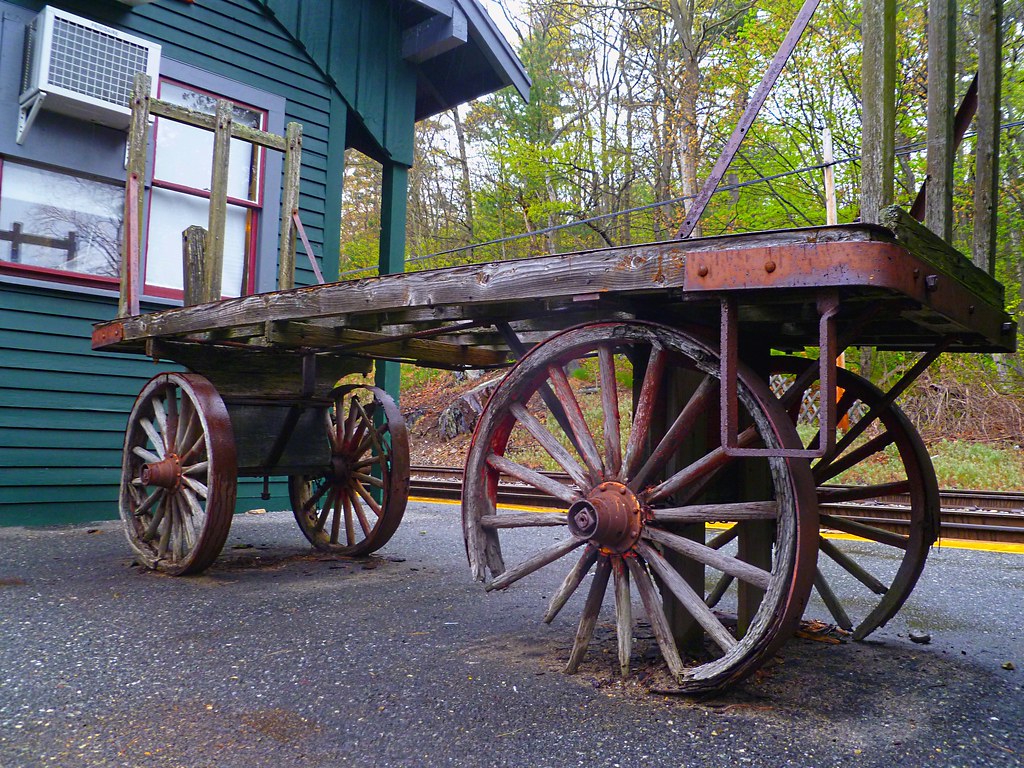This is a horizontal, rectangular image of a very old, weathered wagon or flatbed trailer, likely used in the past for pulling hay or crops behind a horse. The wagon features four wooden-spoked wheels, but they are in disrepair, with some wheels broken and missing pieces. The wood is noticeably rotted, and rust is visible on the metal parts. It sits on a paved driveway or gravel surface. Adjacent to the wagon, to the left side of the image, stands a dark green house with an air conditioning unit mounted in one of the windows. The house has two visible windows. In the background, tall trees with sparse green leaves and a blue sky can be seen, along with a set of railroad tracks running behind the wagon, suggesting the proximity to a potential railroad station.